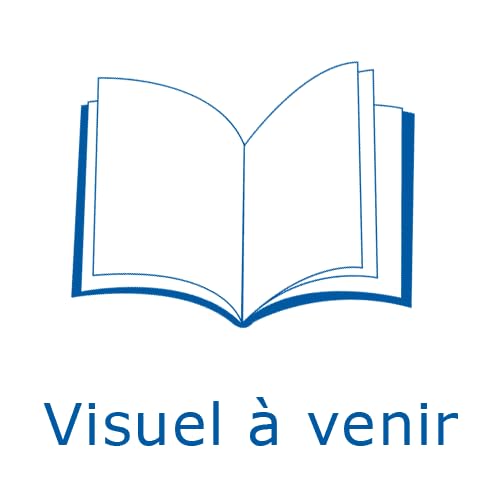The image is a striking advertisement, featuring a close-up of a woman’s pale face, capturing attention with her vibrant, deep red lipstick. Her face, taking up most of the left-hand side and spreading almost across the entire frame, is shown from just below her nose to her bare shoulder, underscored by her light skin. The remainder of the background is a dark red. At the bottom of the image, the word "FEMS" is featured in large, bold letters, with "F-E-M" in red and the remaining "M-E-S" in white, seamlessly blending where the font overlays her neck. The chic, modern style combines elements of photography, illustration, and graphic design, offering a visually compelling and stylish presentation.